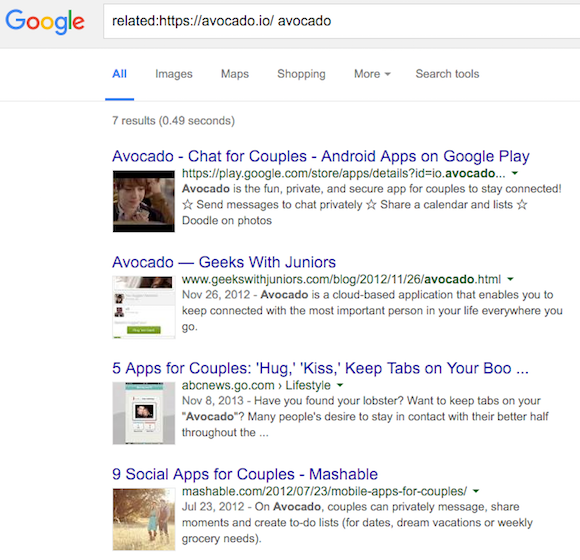The image displays a Google search results page. At the top left, the iconic Google logo is visible with the letters colored as follows: 'G's in blue, 'O' and 'E' in red, the second 'O' in yellow, and 'L' in green. To the right of the logo is the search bar, which contains the query "related:https://avocado.io/avocado". Below the search bar, a set of tabs are present, labeled as "All", "Images", "Maps", "Shopping", "More", and "Search tools". The search returns seven results, which were found in 0.49 seconds.

The first result is titled "Avocado - Chat for Couples - Android apps on Google Play" and includes a snippet that describes Avocado as a fun, private, and secure app for couples to stay connected.

The second result, "Avocado - Geeks with Juniors," describes Avocado as a cloud-based application that helps you stay connected with the most important person in your life wherever you go.

The third result is titled "Five Apps for Couples Hug, Kiss, Keep Tabs on Your Boo" with a snippet that partially reads: "Avocado? Have you found your lobster? Want to keep tabs on your avocado? Many people desire to stay in contact with their better half..." followed by an ellipsis.

The final result, "Nine Social Apps for Couples - Mashable," explains that on Avocado, couples can privately message, share moments, and create to-do lists for dates, dream vacations, or weekly grocery needs.

Each of these entries includes a brief informational blurb indicating that they relate to some type of couples chat or connection application.